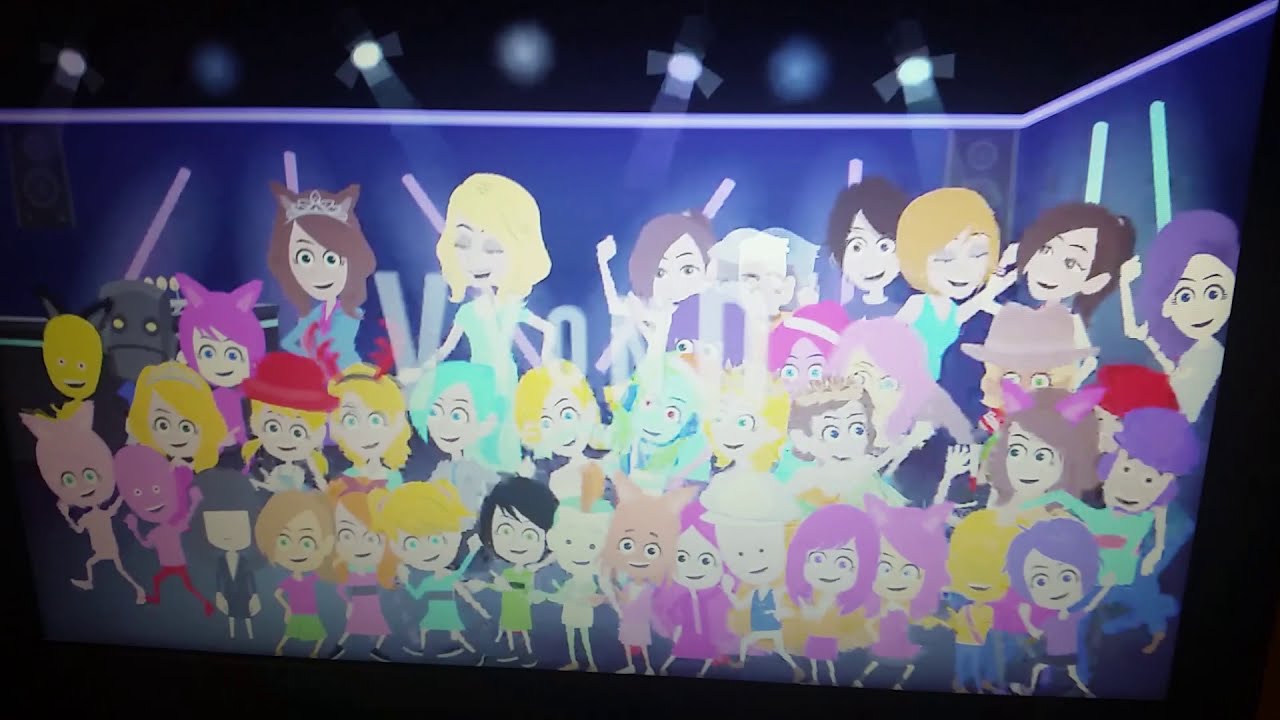The image features a vibrant, cartoonish scene set against an indigo-purple disco-themed backdrop. The central focus is a lively, crowded stage filled with over 30 large-eyed, bobble-headed cartoon characters. These characters, mostly female and sporting a variety of bright outfits and hair colors, range in age from children to adults. They stand closely packed together, with some wearing crowns and cat ears, all appearing happy and engaged with one another. The room, resembling a club, is dark apart from the colorful spotlights and stage lights illuminating the scene from above, emphasizing the party-like atmosphere. The overall composition suggests a dynamic and joyful performance or dance event in a children's show setting.